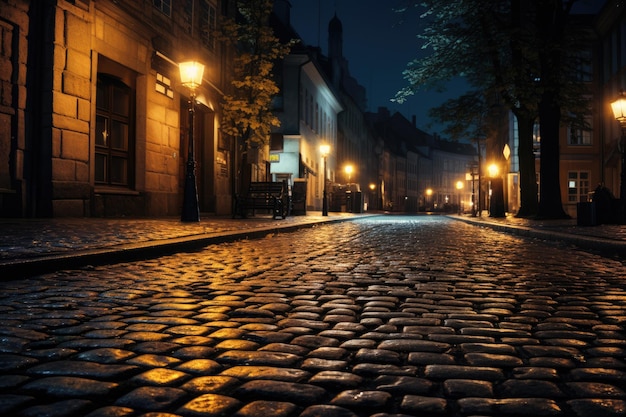The photograph captures a nighttime scene of an old cobblestone street, likely in England, suggested by the architectural style of the sandstone buildings with double doors and large cement stone structures. The glossy, wet cobblestones indicate it has recently rained, reflecting the amber glow of the old-fashioned lanterns that line the street. These black lampposts, casting a warm golden light, illuminate the smooth, weathered road and the cobblestone sidewalks, which are separated by a small raised concrete lip. The road curves gently, with the light growing dimmer as it stretches into the distance. There's a park bench visible on the left sidewalk, adding to the historic charm of the scene. Majestic green trees stand on both sides of the street, their foliage appearing vivid under the streetlamps. The scene is serene and empty, with no people or vehicles in sight, enhancing the tranquil beauty of this timeless city street.